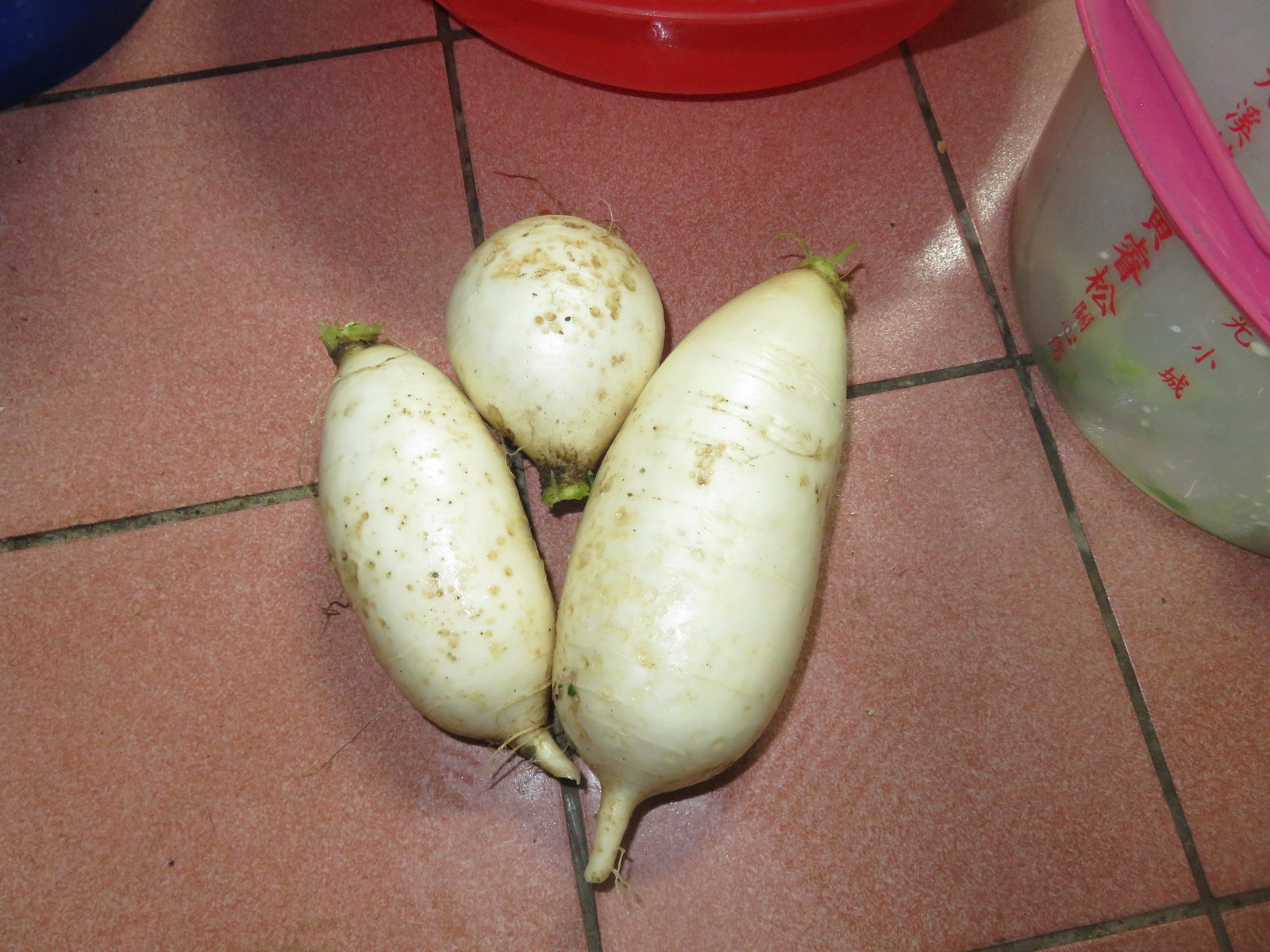The photo depicts a section of a pink tiled floor with dark gray grout between the tiles. In the upper left corner, a small blue object is barely visible, while the very top edge of the picture features a cut-off red object. The upper right corner is marked by a cut-off white and pink object. On the floor are three white vegetables that appear to be radishes. The two on the sides are oblong, with the one on the right being significantly larger. Both have small green nubs at their tops and white elongated tips at their bottoms. The central radish is more globe-shaped and also has a green stalk at one end. The vegetables show some brown dirt spots on their white skin. Additionally, there are plastic pots with red Chinese text along the side in the right portion of the image.